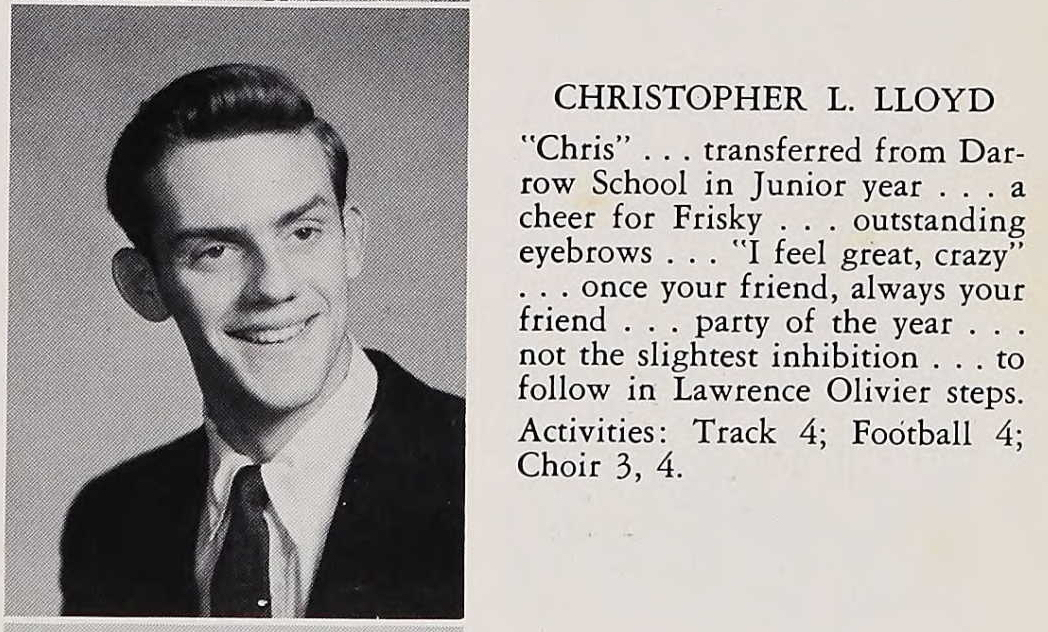The image appears to be a black and white yearbook photograph of a young Christopher Lloyd. He is depicted with his hair slicked back in a style reminiscent of the 1950s or 1960s, smiling keenly off to the lower right of the camera. Christopher is wearing a dark suit and tie paired with a white shirt, emphasizing a professional and polished look typical of high school portraits. The photograph, taken from a yearbook, is grainy and showcases his prominent chin and distinctive eyebrows.

To the right of the image is a detailed blurb under the heading "Christopher L. Lloyd," with "Chris" in quotations. The text reads: "Transferred from Darrow School in junior year, a cheer for Frisky, outstanding eyebrows, I feel great, crazy, once your friend, always your friend, party of the year, not the slightest inhibition, to follow in Laurence Olivier's steps." It also highlights his extracurricular activities: track, football, and choir during his junior and senior years. This blurb reflects his charismatic and spirited personality while hinting at his future aspirations in acting.